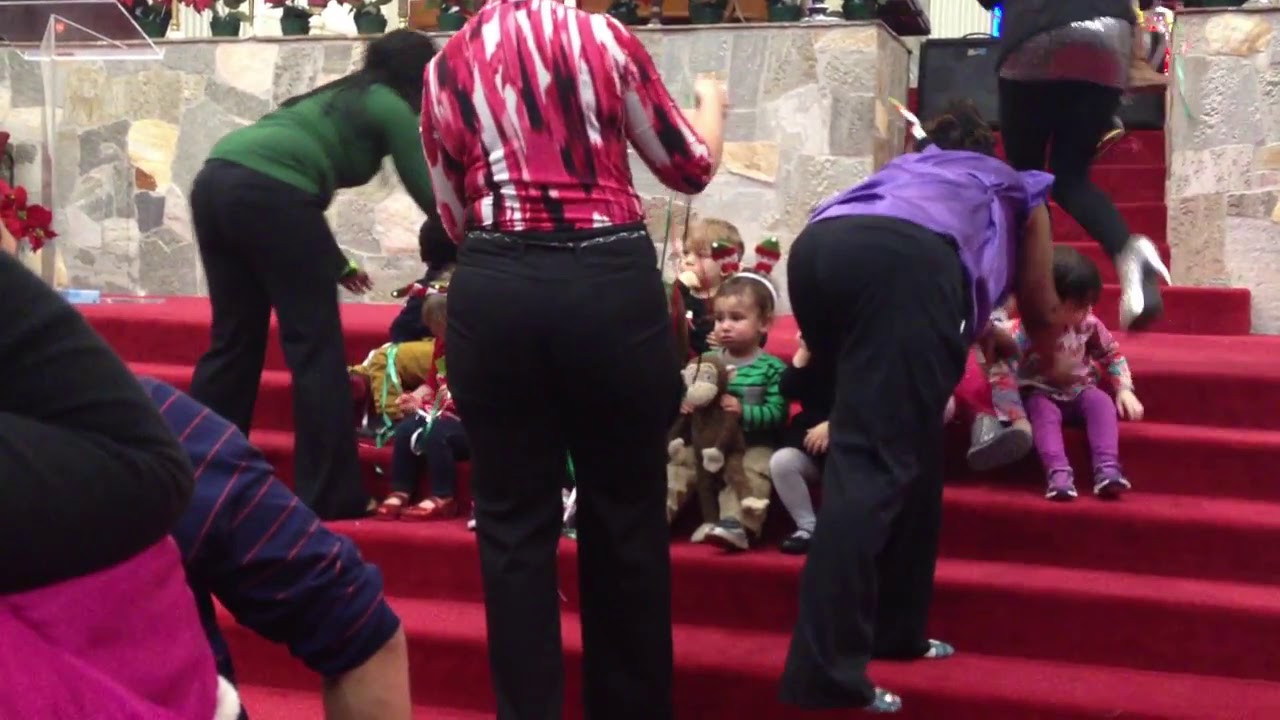This wide rectangular image captures a group of young children, likely toddlers, sitting on red velvet-covered stairs. The stairs span the bottom half of the image, consisting of five steps that lead up to a partial brick counter at the top. The children, dressed in festive Christmas apparel, are surrounded by several adults who appear to be caring for them. 

Three women are prominently positioned in the foreground with their backs facing the camera. In the center stands a woman in black pants and a pink, white, and black shirt. To her left, another woman in a green long-sleeved sweater and black pants is bent over, tending to the children. On the right, a woman in a shiny purple shirt and black pants leans forward, placing a toddler on the step.

Among the children, one little girl stands out. She sits to the left of the woman in the purple shirt, wearing a green and black striped shirt and a white headband with festive elf decorations. The girl clutches a cuddly toy monkey, her expression slightly concerned. The scene suggests a Christmas celebration, possibly within a church, evidenced by the stone effect of the partial wall and counter at the top of the stairs and the overall festive decorations. Additionally, part of an adult's arm is visible in the bottom left corner, slightly out of frame.